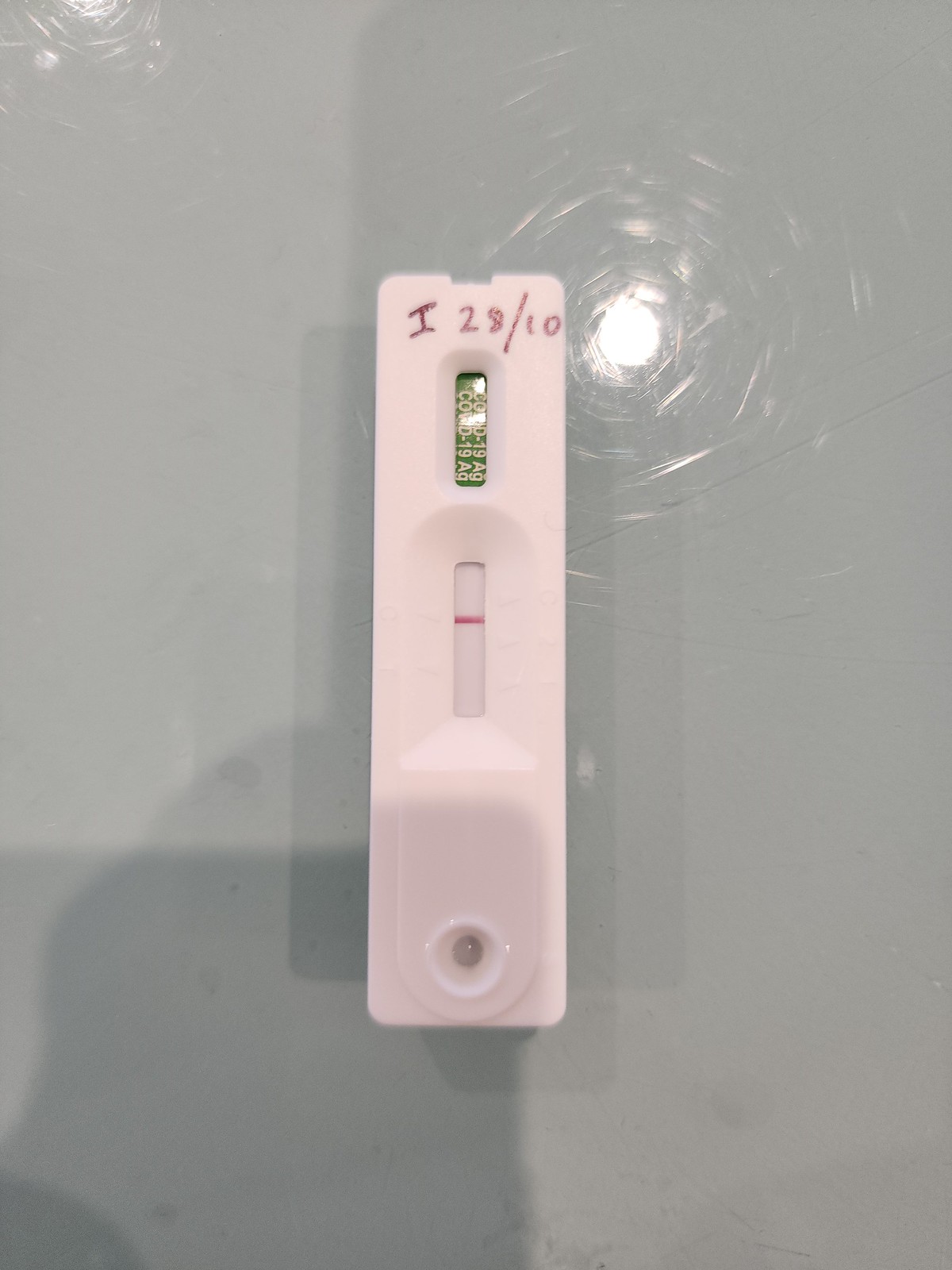The photo vividly captures a COVID-19 antigen test kit placed on what appears to be a protective glass table cover. Beneath the glass, a white cloth is faintly visible. The glass surface shows significant circular scratch marks, clearly reflecting artificial light sources. In the top right corner of the photo, a bright yellow light is reflected, positioned near the test kit. The focus of the image is the rectangular COVID-19 test, which under the lighting appears slightly pink but is likely white. The test kit is marked with "I 28-10," possibly indicating October 28th, although the meaning of "I" remains unclear. The test features two small windows with "COVID-19 AG" labeled twice in the top window. A conspicuous dark red line is visible in the test result window, suggesting a positive result. Below it, there is a circular area designed for inserting the swab, although the swab itself is not present in the photo. Additionally, the image captures the reflection of a hand and the test kit on the glass table.